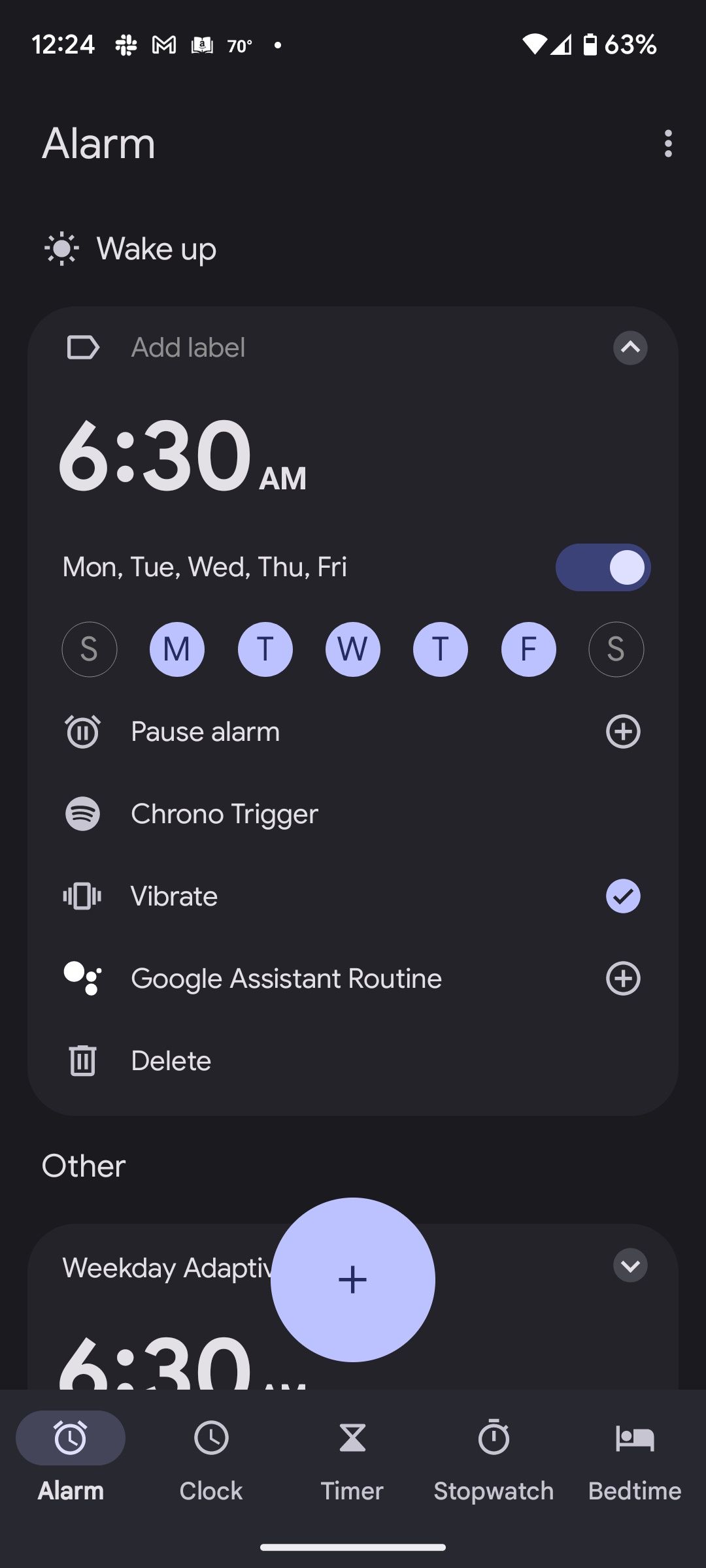This is a detailed description of a mobile screenshot displaying the alarm settings tab with a black background. At the top left corner, "Alarm" is prominently displayed in white letters, while a three-dots icon resides to the right, indicating more options. Just below, a small sun icon is followed by the text "Wake up," both in white.

A section labeled "Add Label" appears next, featuring a drop-down box icon to its right. The alarm time is set to 6:30 AM, presented in large white numerals. The section beneath showcases the days of the week: Monday, Tuesday, Wednesday, Thursday, and Friday, each accompanied by a toggle switch on the right. The toggle switch is turned on, indicated by a blue background within the bubble.

Further down, a row displays the abbreviated days of the week, "SMTWTFS," with Monday through Friday encircled in blue to denote they are selected. Following this, the option "Pause Alarm" is listed with a plus icon to its right. Below are additional settings including "Chrono Trigger," "Vibrate," "Google Assistant Routine," and "Delete."

Finally, a large, centered plus sign icon in a circle is located at the bottom of the screenshot.